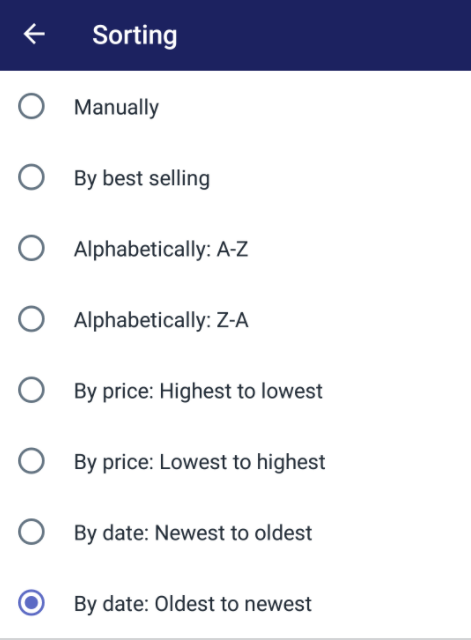A detailed description of a website's sorting menu, likely from a shopping site such as Amazon, is depicted in this image. The sorting options are presented in a clean, user-friendly interface. Dominated by a dark navy background, the menu's title, "Sort," is prominently displayed in white within a horizontal dark blue bar. To the left of this title, a white arrow icon serves as a back button.

Beneath the title, a series of sorting options is listed, each accompanied by a circular radio button for selection. The options are as follows:
1. Manually
2. Best Selling
3. Alphabetically: A-Z
4. Alphabetically: Z-A
5. Price: High to Low
6. Price: Low to High
7. Date: Newest to Oldest
8. Date: Oldest to Newest

The radio button next to the "Date: Oldest to Newest" option is filled in, indicating it is currently selected. Despite the lack of explicit branding, the structure and choices strongly suggest that this sorting menu is from a shopping site, most likely Amazon.